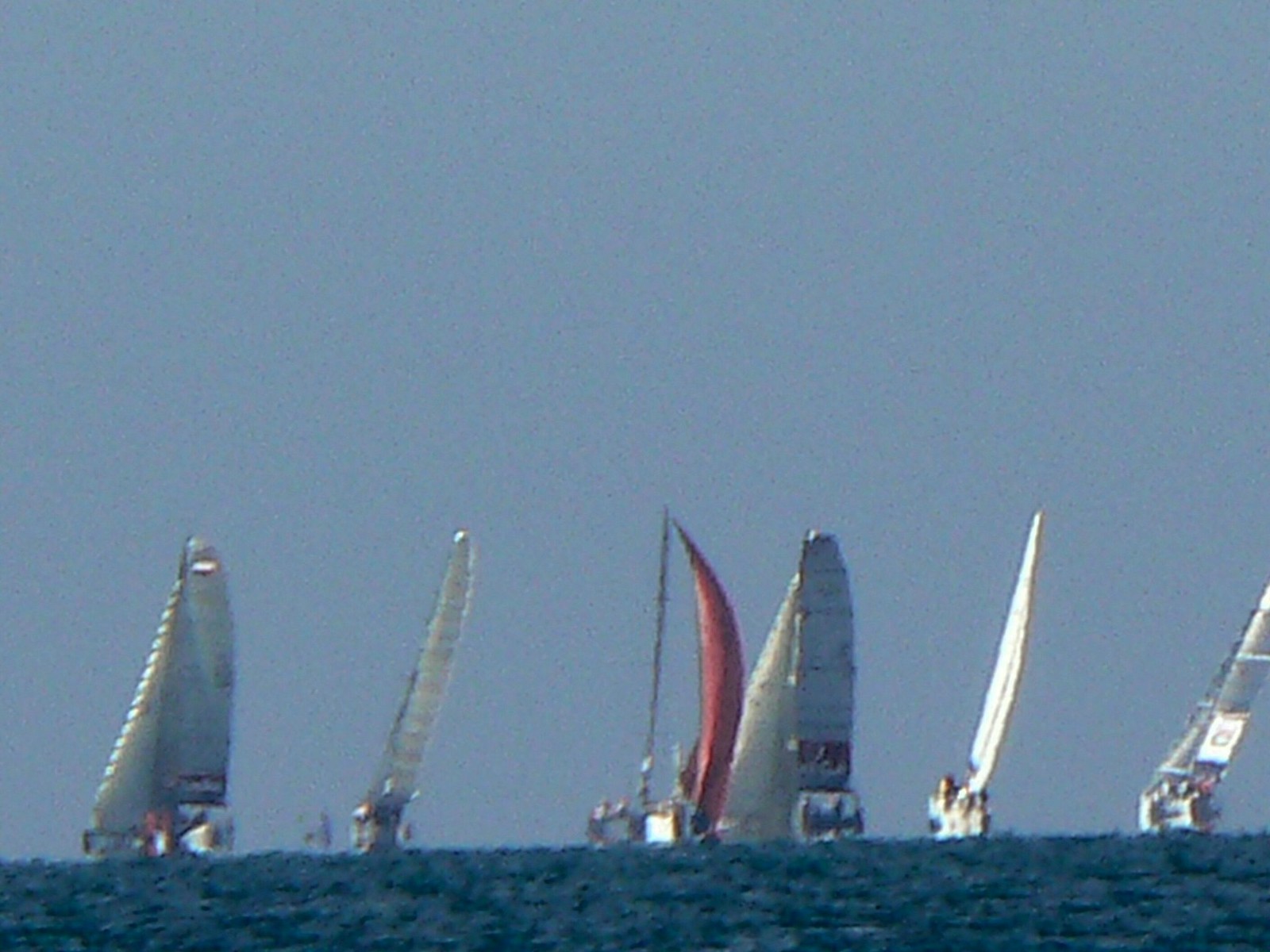In this slightly blurry photograph, six small sailboats are lined up in a row, creating the impression of a potential race on the open ocean. Each boat is structurally similar, with large sails in comparison to their size, and most feature white sails with subtle differences in color and design. The third boat from the left stands out with its bright red sail, which is tethered by a string at both the top of the sail and the bottom center of the boat. The boat on the far bottom left has a notably triangular sail and a small rudder on its right side for wind direction. The boat furthest to the right has a distinctive logo on its sail, though it is not clearly identifiable. The ocean's bright blue hue contrasts with the light gray tone of the sky, which occupies the majority of the background and is depicted without any clouds. Despite the image's pixelation and slight blurriness, there are visible waves in the water, enhancing the dynamic feel of the scene.